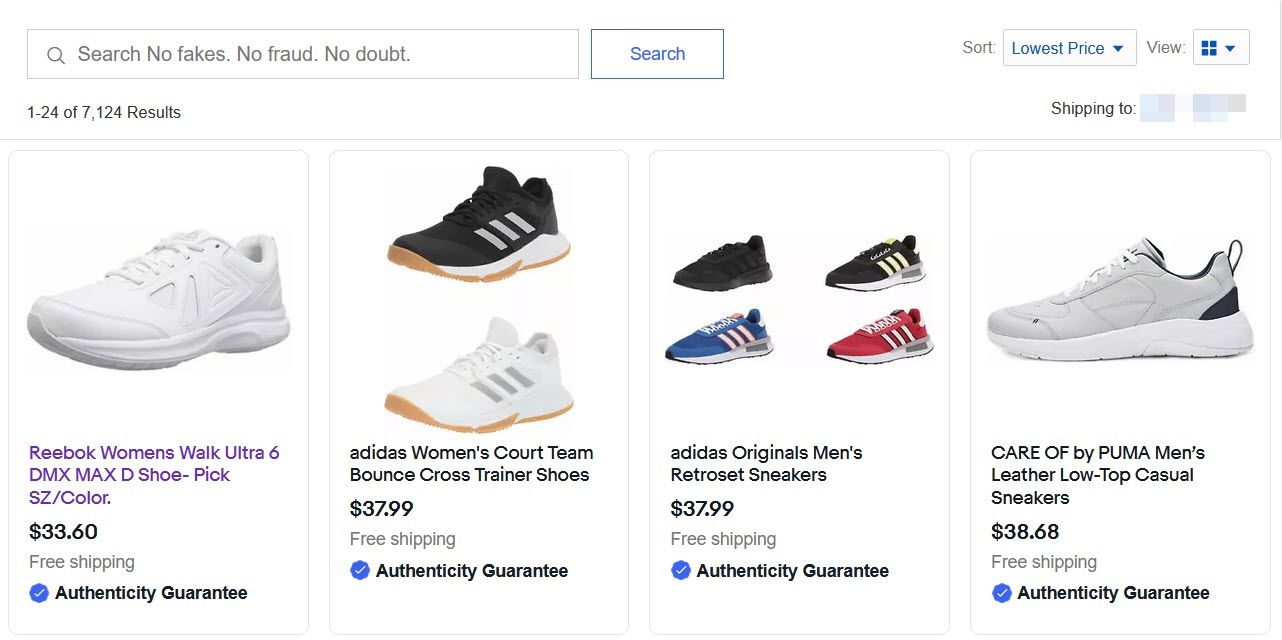The image depicts a webpage, likely from eBay or a similar online marketplace, showcasing search results for sneakers. The title displayed above the search bar prominently states, "No Fakes, No Frauds, No Doubt." Featured on the page are four pairs of sneakers, each accompanied by their price, a free shipping icon, and an authenticity guarantee badge. The listed sneakers include:

1. **Reeboks Women's Walk Ultra 6 DMX Max D Shoe** – Priced at $33.60.
2. **Adidas Women's Court Team Bounce Cross Trainer Shoes** – Priced at $37.99.
3. **Adidas Original Men's Retro Set Sneakers** – Priced at $37.99.
4. **Care Of by Puma Men's Leather Low Top Casual Sneakers** – Priced at $38.68.

All items offer free shipping and come with a guarantee of authenticity. The page indicates that these are just four of a total of 7,124 available sneaker results, suggesting a vast selection on the platform, likely aligning with eBay's format.